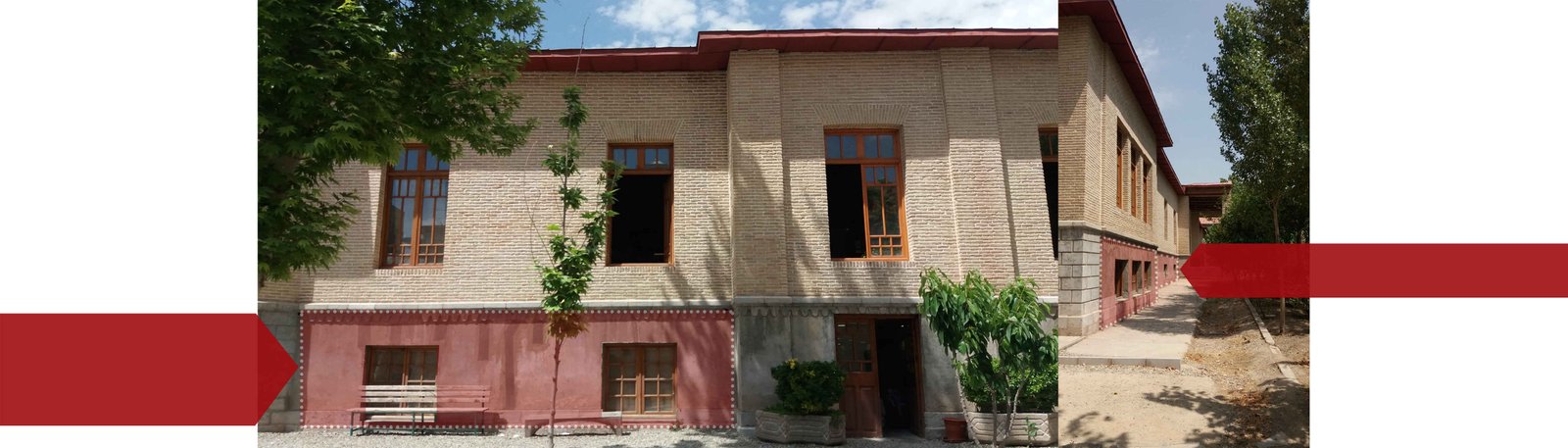This detailed image displays two juxtaposed photographs of a two-story building forming a panoramic view. The larger photograph on the left, occupying approximately two-thirds of the composition, showcases the front façade. The top half of this building is constructed with light tan bricks, featuring three rectangular windows framed with brown wooden grids. A flat roof caps the building, beneath which, the first story diverges—two-thirds covered in red brick with windows and doors, and one-third in gray stone where a small tree is positioned. Adjacent to the building, a park bench and a few potted bushes are visible against the red-bricked section, while the gray area reveals another small tree near the doorway. The photograph includes a portion of a vibrant blue sky dotted with clouds and trees in both the upper left and lower right corners.

The adjacent image on the right highlights a side perspective of the building, revealing a walkway with trees and a dirt path. Red arrows prominently point inwards from the left and right sides of the images, with a shorter, thicker arrow on the left directing attention to the first story's red brick area, and a longer, thinner arrow on the right marking another red section on the building. The overall scene, set against a plain white background without visible borders, conveys an outdoor setting suggestive of an office environment.